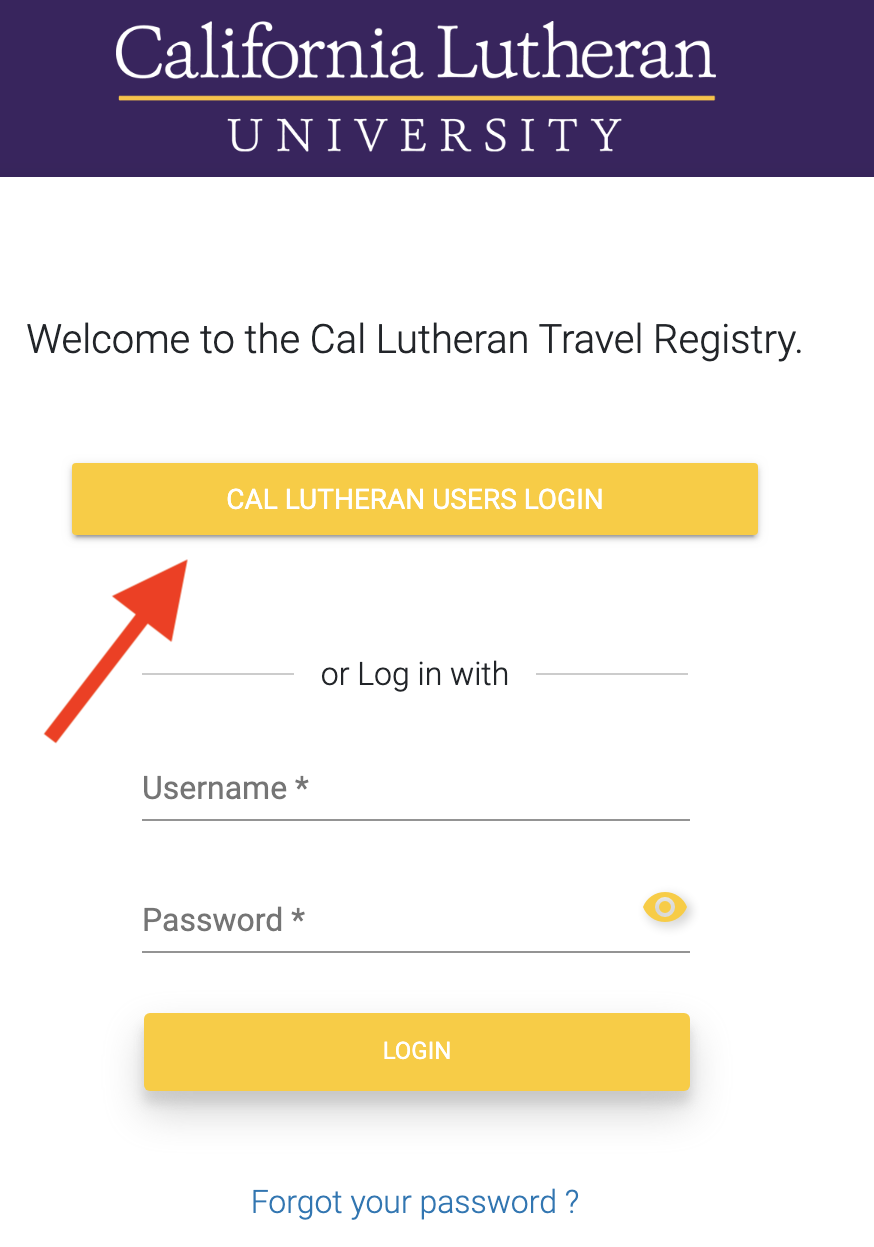The image depicts the login window for California Lutheran University, set against a predominantly white background. At the top of the window, a royal purple header displays the text "California Lutheran" in white, followed by a thin yellow line beneath it. Directly under the yellow line, the word "University" is printed. Below this header, a white expanse introduces the login section with the greeting, "Welcome to the Cal Lutheran Travel Registry." 

Centered below this welcome message, a prominent yellow horizontal button with white text reads, "Cal Lutheran Users Login." A large red arrow points directly at this button, drawing attention to it. Further down, the text "or login with" suggests an alternative method for accessing the system via a username and password.

In this section, there are two input fields: the first for the username and the second for the password, the latter featuring a small yellow eye icon on the right side to toggle password visibility. Below these text boxes, another yellow button labeled "Login" invites users to proceed. At the very bottom of the image, the option "Forgot your password?" is provided in blue text for users who need to recover their login credentials.